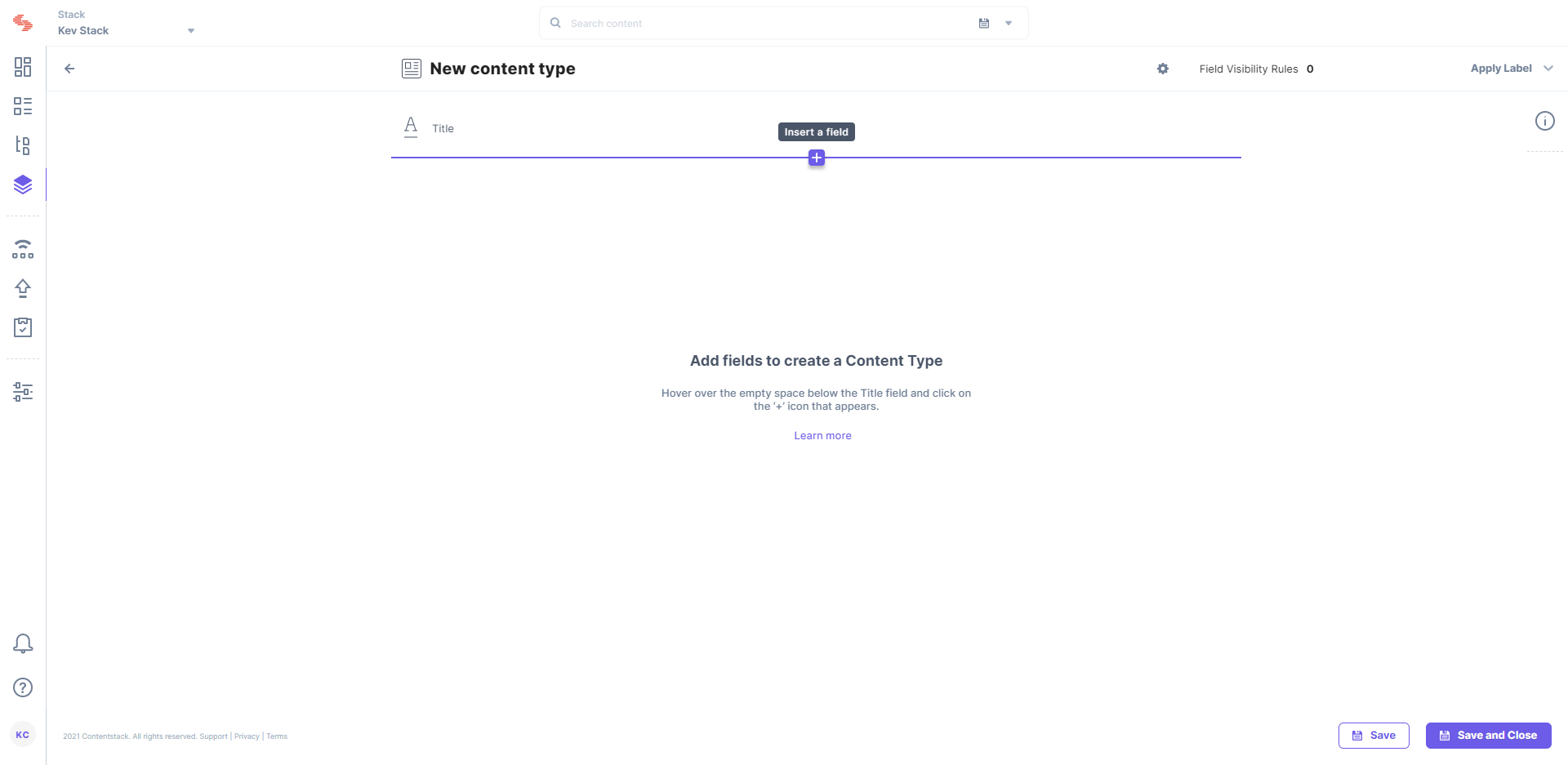This screenshot displays the interface of a web application named Stack, identifiable by its red emblem and the "Stack" logo positioned in the upper left corner. The logo is accompanied by the text "KEV Stack KEV Stack." The main purpose of this web app appears to be for creating and managing pages for websites or apps, featuring various templates, settings, and functionalities.

In the middle section of the screen, there's a headline reading "New Content Type" accompanied by a small icon resembling a newspaper. Below this, a field labelled "Title" is visible, next to which is a character "A" with an underline, indicating the user should begin typing the title of their new page in this space.

Further down, an option labeled "Insert a Field" allows users to add different fields to their content type. A note beneath this reads: "Add fields to create a content type. Hover over the empty space below the title field and click on the plus icon that appears." There is also a "Learn More" button for additional guidance.

At the top of the interface, there's a section titled "Field Visibility Rules" currently showing zero rules, and an "Apply Label" option next to an eye icon enclosed in a circle, likely signifying visibility settings.